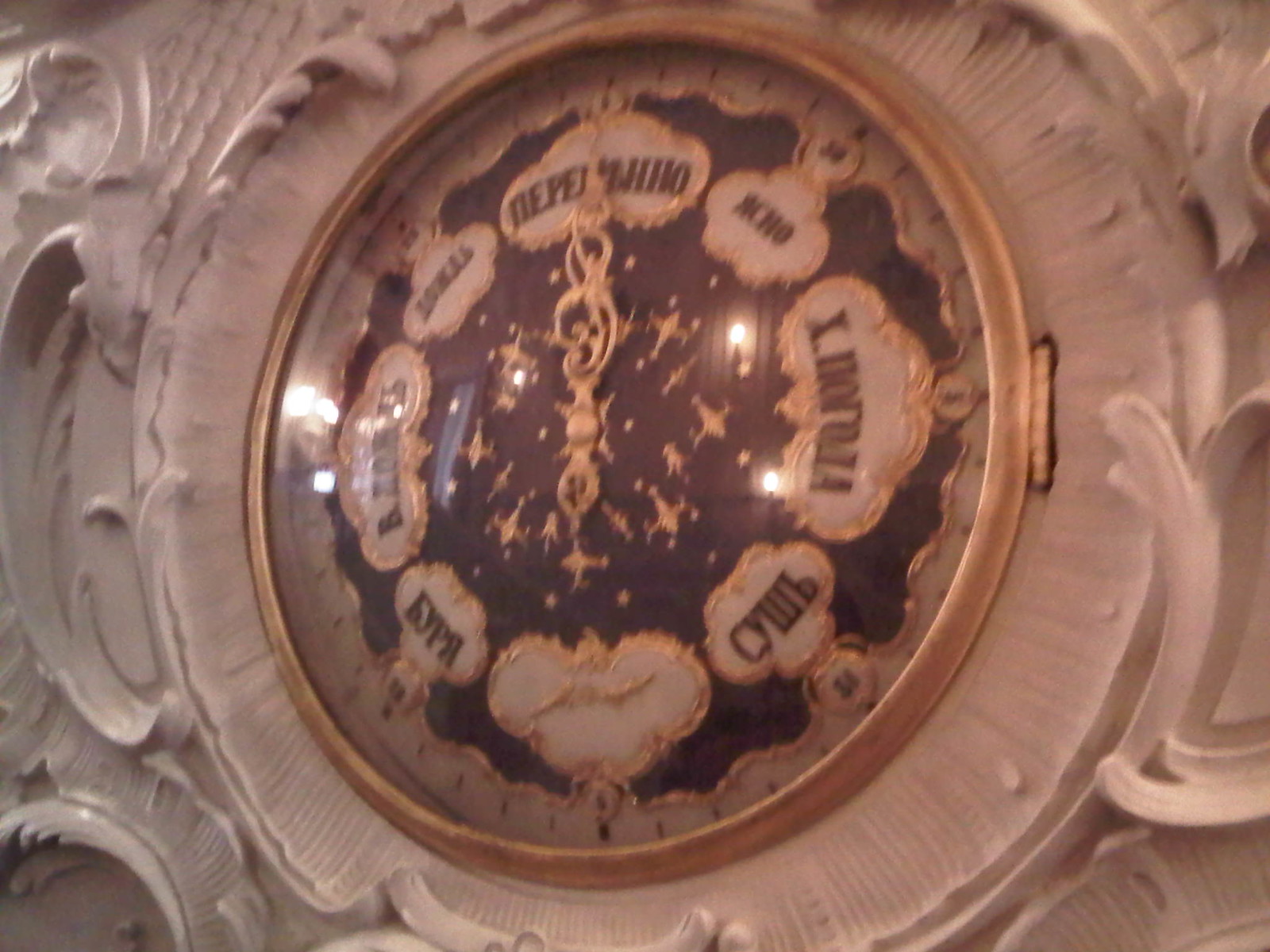In this slightly blurred photograph, there is an elaborate, antique clock displayed. The timepiece is strikingly ornate, with its hands set precisely at the 12 o'clock position. The clock's face features a dramatic black background lavishly decorated with intricate gold inlay. Surrounding the face, Roman numerals denote the hours, although the exact details of the inscriptions are faint. Adding to its unique design, the clock is embellished with motifs of stars and possibly zodiac signs.

The clock hands are gold, complementing the opulence of the design. This exquisite piece is mounted on a prominent, large, white wooden plate, adding to its striking appearance. The juxtaposition of the black and gold clock against the white background enhances its visual impact. The overall aesthetic is both rare and captivating, making it a truly remarkable timepiece. Both clock hands meeting at the 12 o'clock mark underline the elegance and precision of this extraordinary object.